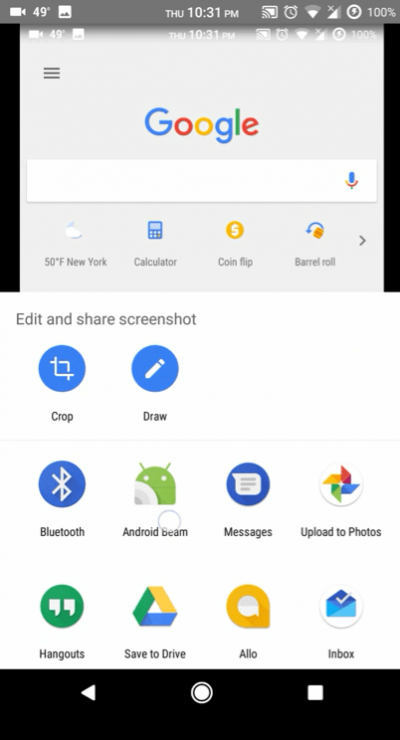**Detailed Smartphone Screen Description:**

A detailed screenshot of a smartphone screen features a variety of elements and icons, with a prominent blow-up section highlighting specific details. The smartphone screen is outlined in dark gray at the top and black on the sides and bottom. At the top of the screen is a status bar displaying white font text that indicates the battery is 100% charged and the current temperature is 49 degrees. Additionally, it shows the time as 10:31 p.m on a Thursday.

The main part of the screen is a Google search page. The familiar Google logo with its multicolored letters is situated above a white search bar. To the right of the search bar is a microphone icon, indicating the option for voice-to-text input. Beneath the search bar, the temperature is displayed as 50 degrees Fahrenheit in New York. This section is accompanied by a row of icons, including a calculator, a coin flip feature, and a 'barrel roll' option, with an arrow pointing to the right for additional options.

Overlaying the top section of the screen is a white rectangular pop-up banner that extends across the screen, labeled "Edit and share screenshot." It features tools including a blue circle with an overlapping L-shaped crop icon labeled "Crop" and another blue circle with a white pencil draw icon labeled "Draw."

Below the pop-up, there is a row of sharing options: 
- **Bluetooth:** Represented by a blue circle with the Bluetooth logo.
- **Android Beam:** Featuring the green Android robot icon.
- **Messages:** Indicated by a blue circle with a chat speech bubble containing lines.
- **Upload to Photos:** Displayed with the Google Photos pinwheel icon.

Another row of icons includes:
- **Hangouts:** Shown as a green circle with white quotation marks.
- **Save to Drive:** Represented by a Google Drive triangle in Google's signature colors.
- **Allo:** Another text app indicated by a yellow circle with a white speech bubble.
- **Inbox:** Displayed as a white circle with a blue envelope logo.

At the bottom of the screen, there is a black navigation bar with the standard icons: a left-pointing arrow, a circle in the middle, and a square on the right.

Overall, this detailed caption captures the comprehensive layout and various features of the depicted smartphone screen.